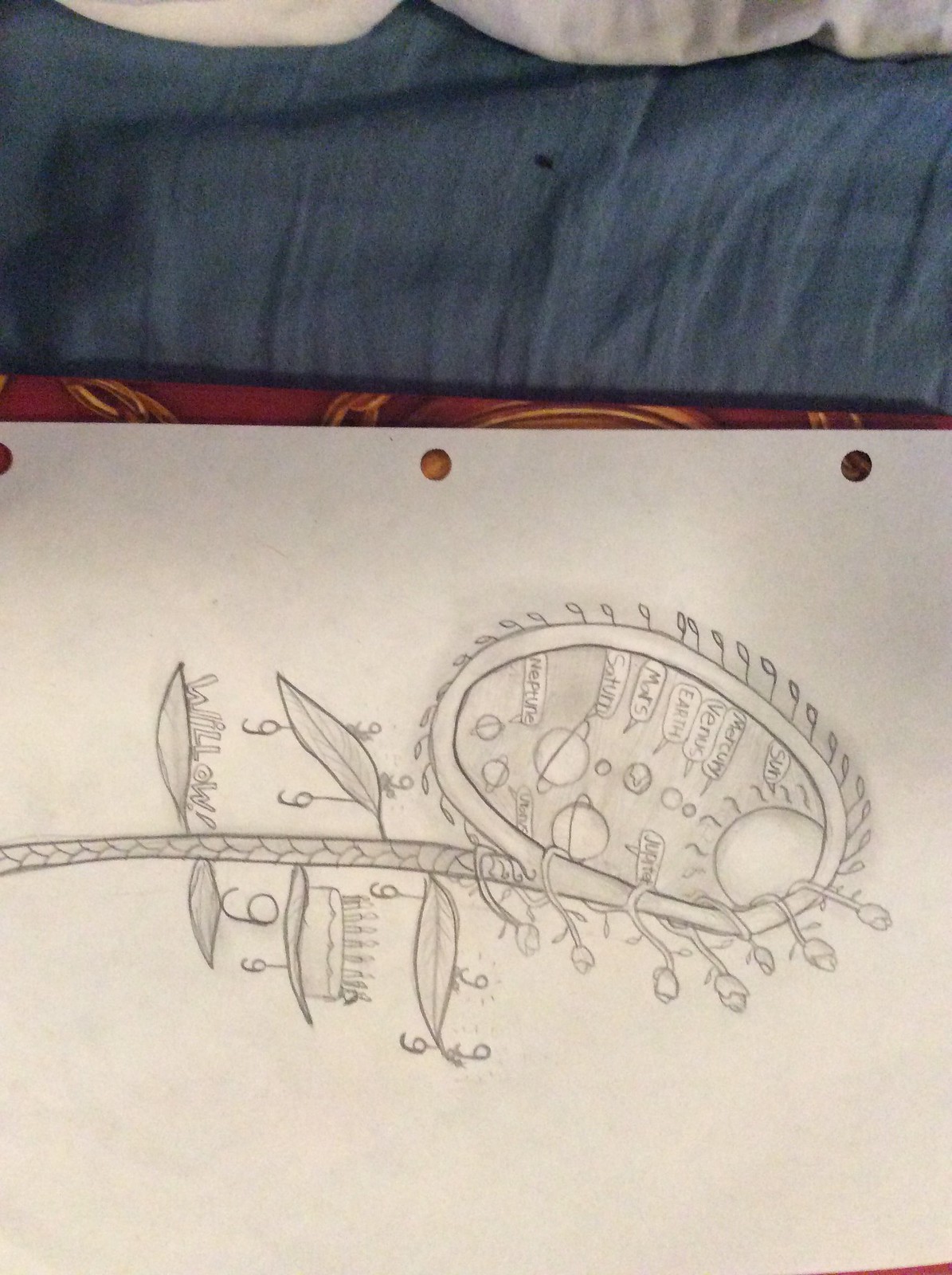A detailed and descriptive caption for the given image could be:

"In this intricate sideways sketch, presented on paper, the design prominently features a floral motif. The sketch, primarily rendered in gray, displays a singular vine adorned with regular patterned lines. Leaves sprout from this vine, with three leaves on the right and two on the left, each leaf having a number nine figure extending from it. At the top of the vine, smaller tendrils intertwine and culminate in a circular structure, embellished with shapes reminiscent of musical notes on the left side of the 'flower.' The image needs to be rotated 90 degrees clockwise for proper viewing. Three punch holes line what appears to be the top edge of the sketch from this angle, indicating the paper's orientation. The sketch rests on a surface partially visible at the bottom, showcasing hints of brown and gold, while a blue background subtly frames the upper portion of the image, adding contrast and depth to the artwork."